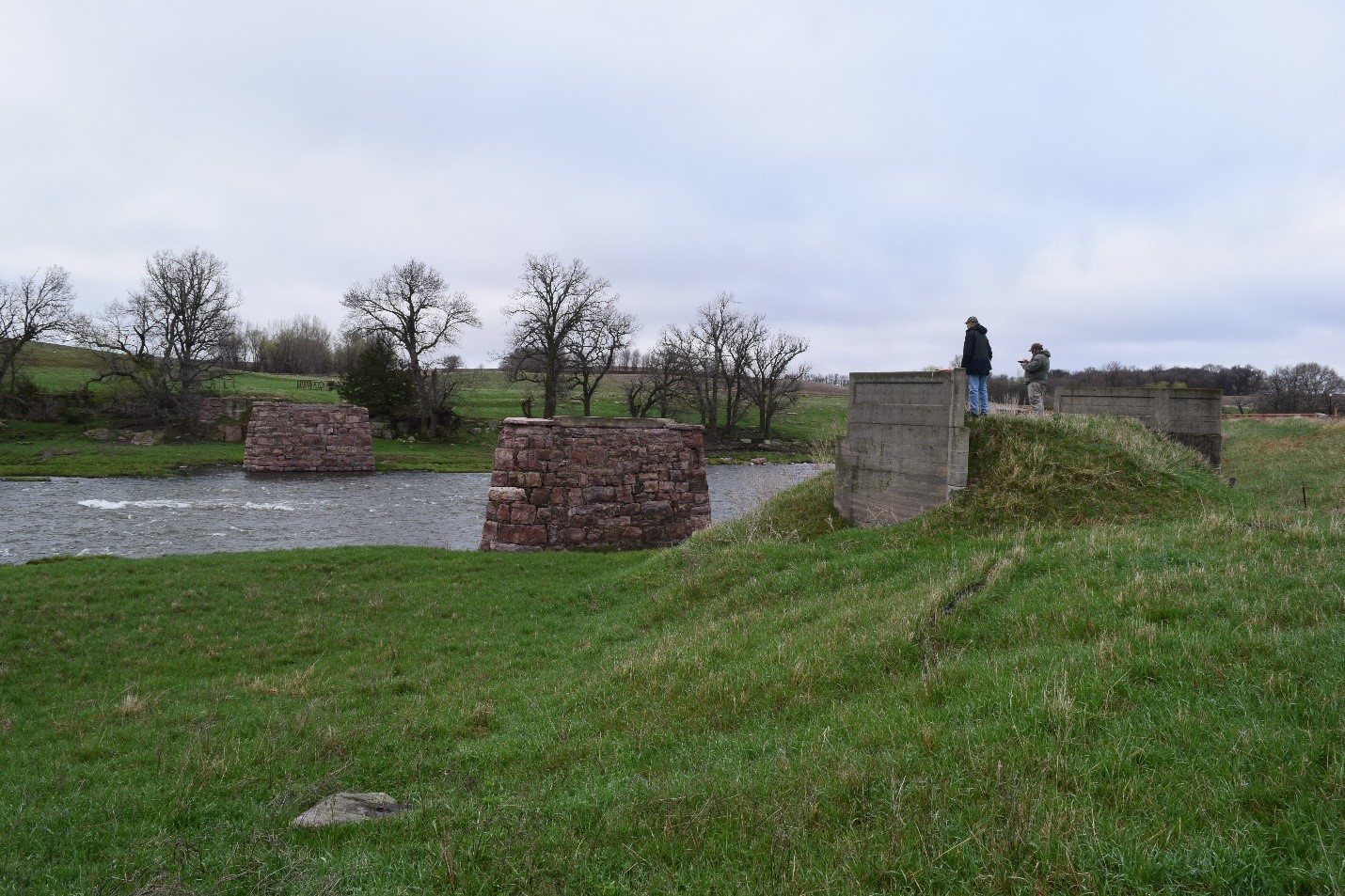The photograph captures a serene outdoor setting under a mostly cloudy sky with hints of blue peeking through. The scene features a small body of water, possibly a river or large stream, flanked by the remnants of an old stone bridge. The stone columns on either side of the water once supported the bridge and are made of imposing, layered stone still standing strong despite the bridge's absence. In the foreground, there's green grass with touches of brown, leading up to a grassy mound where two people—likely men—stand near additional stone structures that could have marked the bridge's approach. The background showcases a hill covered in green grass and a cluster of bare trees, suggesting it is fall or winter. The overall atmosphere is somewhat muted, with a subdued color palette and an overcast sky, lending a timeless, nostalgic feel to the landscape.